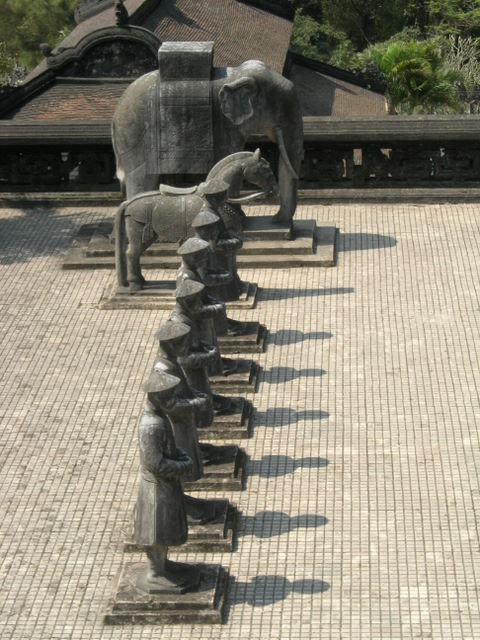In this detailed aerial view photograph, we see an impressive lineup of intricately crafted stone statues, each standing on pedestals on a tiled surface made of small square concrete tiles. Prominently featured is an imposing statue of an elephant at the forefront, distinguished by a box shape on its back draped with fabric flowing down its sides and back. Directly next to the elephant stands a saddled horse adorned with armor.

The scene continues with six identical statues of men, meticulously arranged side by side in a row. These statues are dressed in knee-length tunics and boots, each holding their hands in front of them and donning disc-shaped hats reminiscent of Asian rice field workers' hats. 

The setting appears to be an ancient temple or a sacred site, with the background revealing the roof of another building constructed in a traditional Asian architectural style, partially obscured by lush green foliage. All these combined elements create a visually captivating and culturally rich tableau.